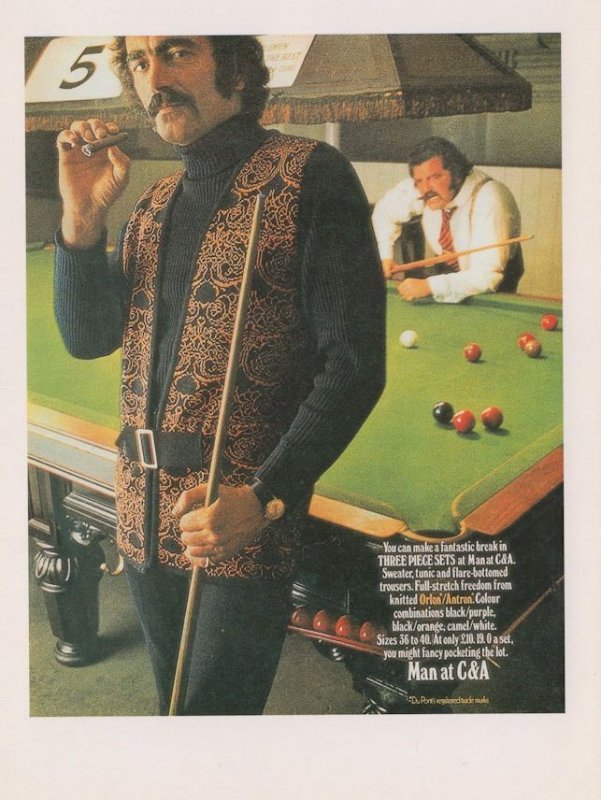This picture, slightly blurred and with a vintage feel possibly from the 1970s, appears on a poster board showcasing a man playing snooker while smoking a cigar. He is prominently dressed in an ornate dark vest adorned with a red or gold tapestry design, paired with a belt and black long sleeves. His left hand holds a cue stick as he faces the camera. 

Behind him stands another man in a white long-sleeve shirt with a red tie and suspenders, also holding a cue stick. Both men exude an air of toughness, resembling pool sharks, and they appear to be of Italian descent. 

The pool table, central to the scene, is a well-crafted, heavy-duty piece that speaks to an earlier era's craftsmanship, and it’s illuminated by a light fixture above it. In play are the distinct red balls of a snooker game, a white cue ball, and a black ball, indicating this is a game for skilled players. 

At the bottom right of the image, there is text that reads, "Man at CNA," which seems to be part of a larger blurb stating, "You can make a fantastic break in three-piece sets at Man at CNA." Additional details about the fashion include different fabric combinations in black and purple, and size information ranging from 36 to 40, suggesting that this image might be an old fashion magazine promoting men's formal wear.